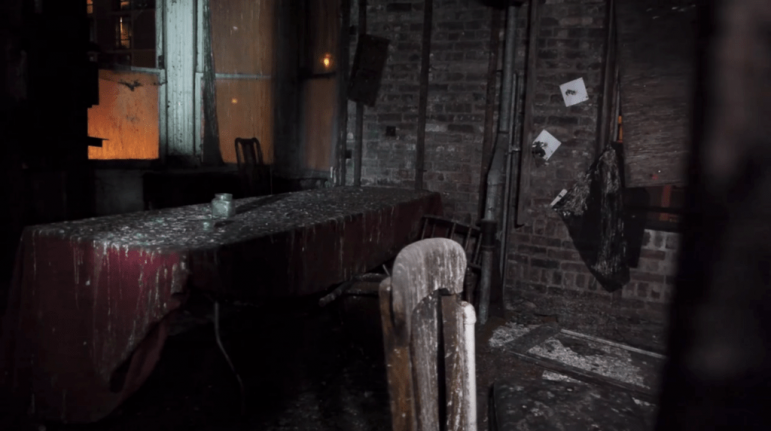The photograph depicts a deteriorating room with an industrial ambiance, characterized by its brown brick walls that suggest an underground or secluded setting. The space is cluttered with dirt and debris, reinforcing its neglected state. Prominently featured in the center is a table draped with a burgundy tablecloth, notably marred by white paint stains. Surrounding the table is broken, worn-out wooden debris, adding to the room's abandoned atmosphere. An orange glow filters through a window, casting a haunting light that contrasts starkly with the room's disarray. The overall scene evokes the image of a forsaken storefront or restaurant, left to decay over time.